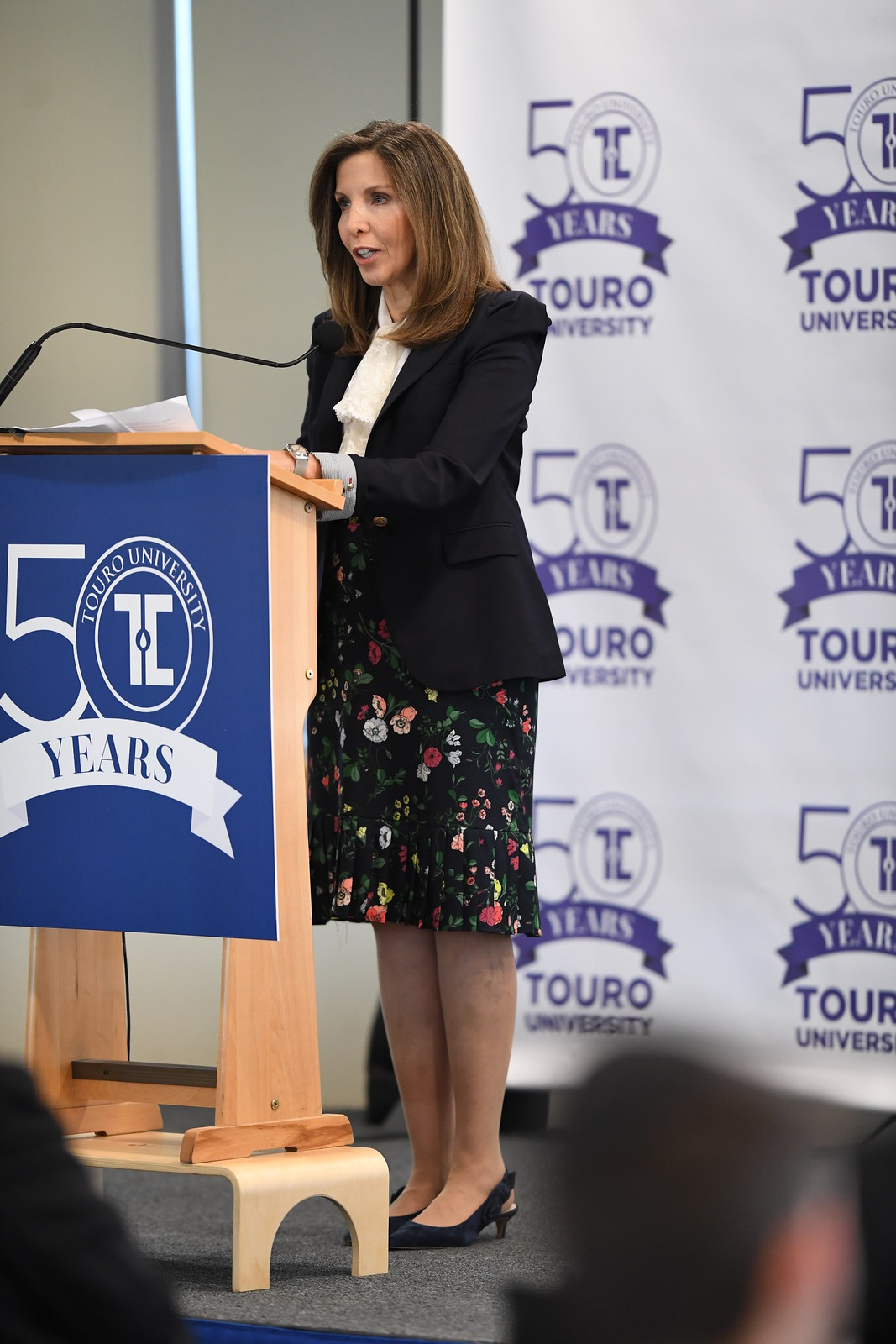In this image, a middle-aged woman with shoulder-length brunette hair, highlighted in brown, stands at a wooden podium positioned on a small wooden stool to elevate it. The podium features a blue sign with the number "50" in white, and within the zero, it reads "Touro University." Below it, a white banner with blue text states "years." The woman, centrally positioned in the image, is addressing a crowd and speaking into a microphone, with papers spread out in front of her. She is dressed in a black blazer, a white blouse, a knee-length floral skirt, and black slingback heels. Behind her is a large white poster repeating the "50 years Touro University" emblem. The setting appears to be indoors on a carpeted surface, and the scene suggests an event celebrating the 50-year anniversary of Touro University. The prominent colors in the image include black, blue, gray, light brown, pink, purple, and white, providing a formal and celebratory atmosphere.